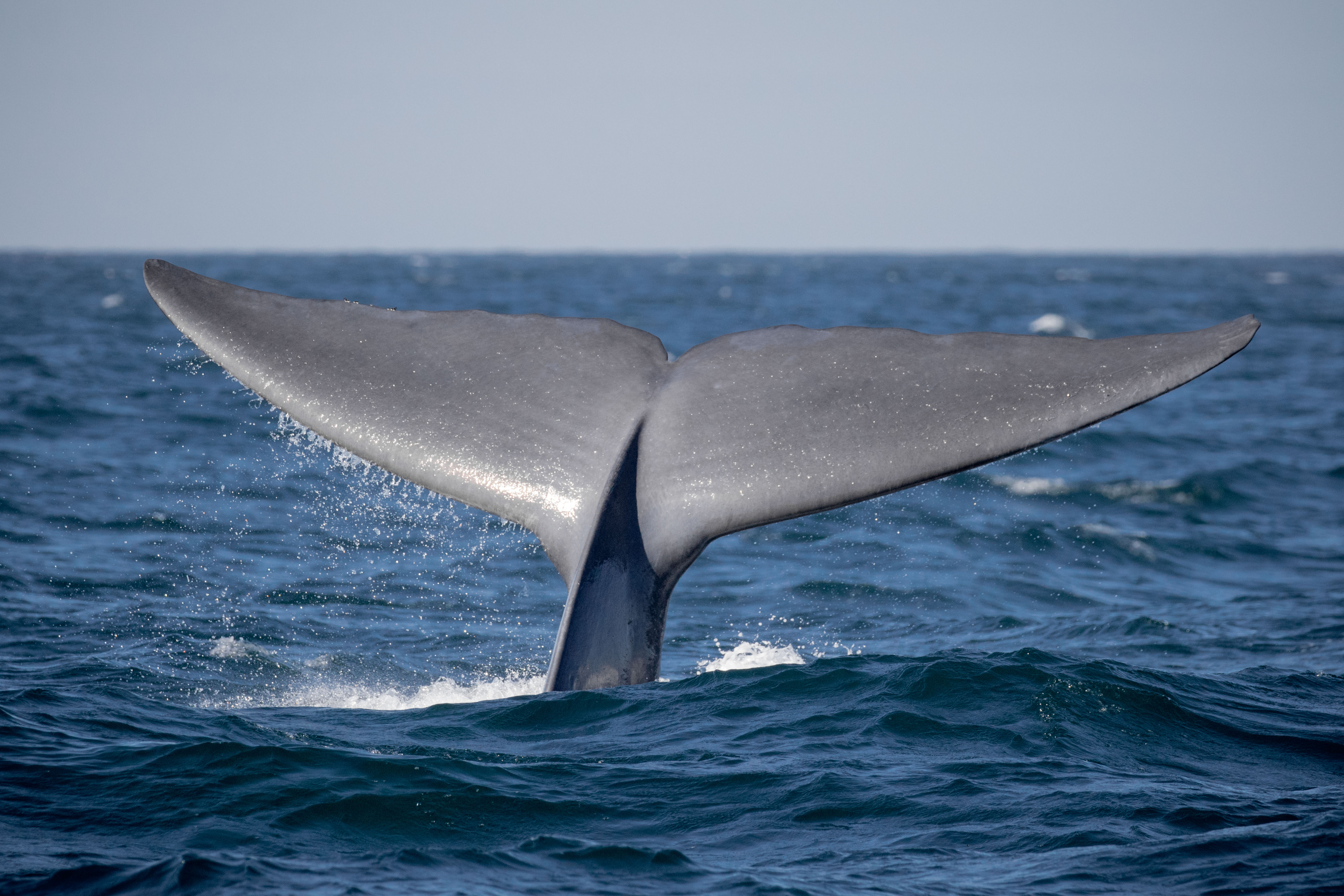A compelling photo captures the majestic moment of a gray whale's tail, or flukes, gracefully slicing into the calm, dark waters of the ocean. The whale is diving, likely aiming for a deeper, more fruitful layer of the sea. No land disrupts the vast expanse of blue, indicating that this scene is set far offshore, possibly taken from a boat. The smooth horizon is dominated by a cloudy sky, adding a serene backdrop to the spectacle. Tiny caplets of wind-driven waves scattered across the water surface lend a gentle texture to the scene. Tiny droplets of water glisten on the whale's tail, casting a hint of sparkle as they catch the light, emphasizing the tail's elegant descent. The combination of a slightly wavy sea and the distinctive elements of the whale's dive makes this image a breathtaking capture of marine life in its natural habitat.